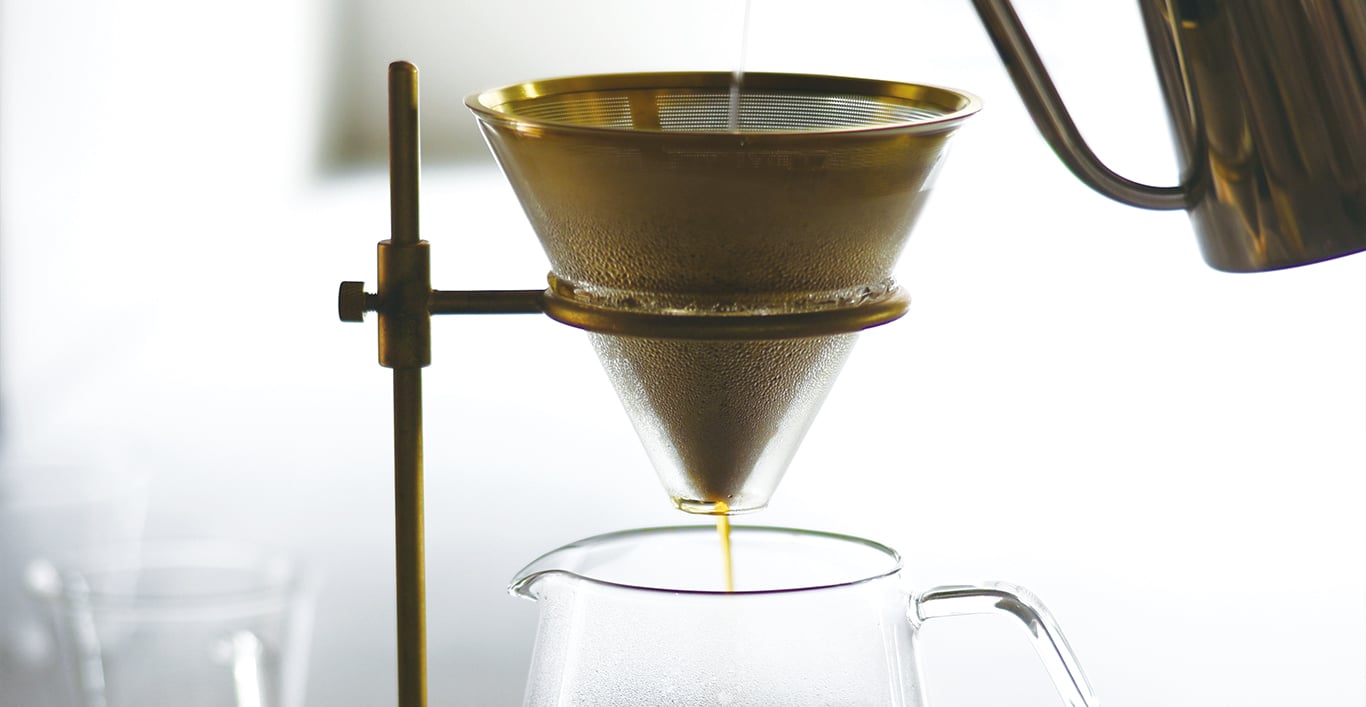This close-up photograph vividly captures the process of making coffee using a manual drip coffee device. At the center of the image is a brass brushed funnel with an integrated mesh filter, securely held in place by a brass stand consisting of rods and a tightened screw, creating a stable base for the funnel. Clear water is being poured from a seen-but-partially-out-of-frame brass kettle into the top of the funnel. As the water passes through the filter, it transforms into a rich, amber coffee, which drips into a clear glass pitcher positioned below. The background is softly blurred, highlighting the sharp foreground details of the brewing process. Additional out-of-focus elements include several glass jugs and a framed picture on a white wall, adding context to the brass and glass textures that dominate the image's color palette.